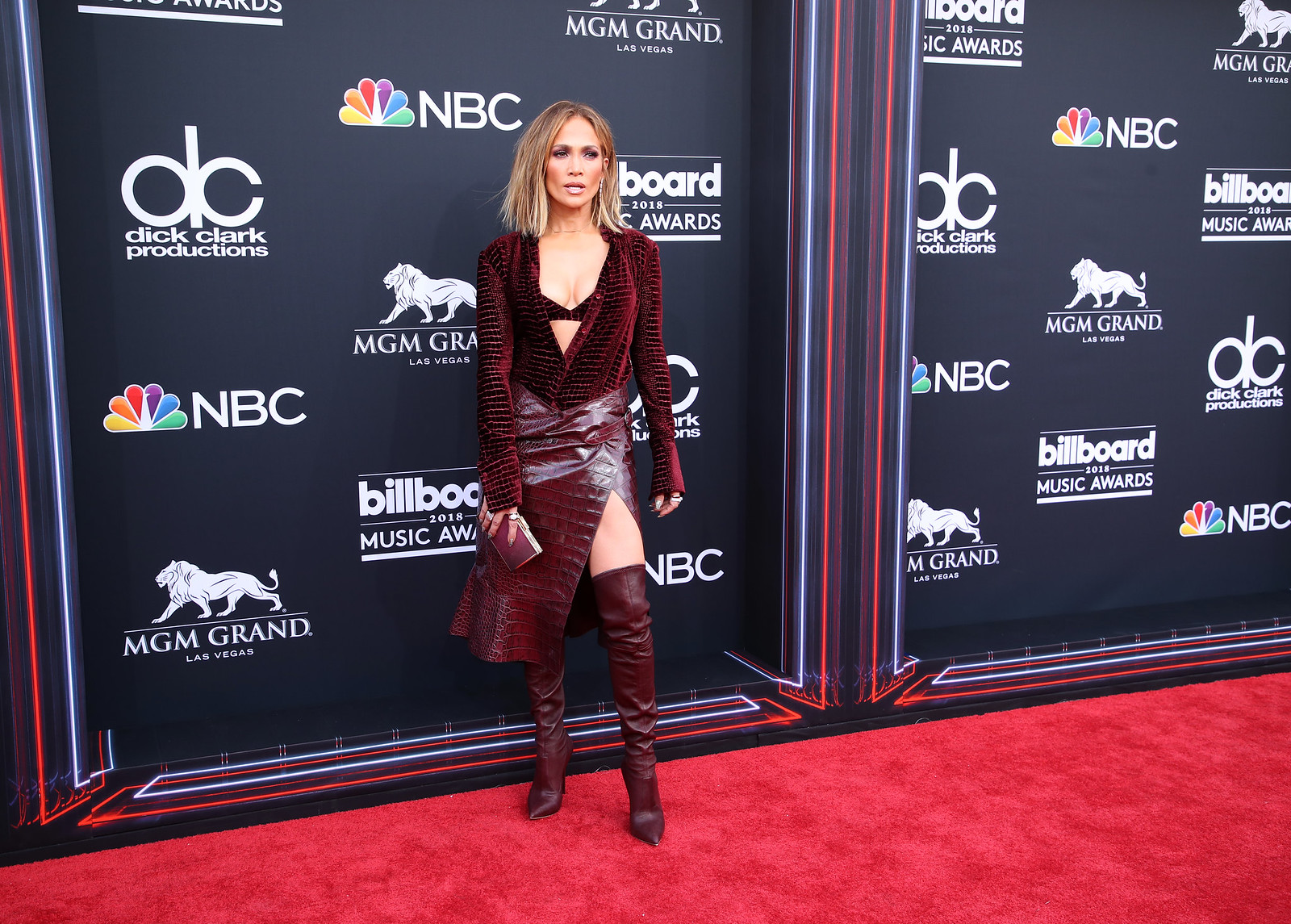This image features Jennifer Lopez gracing the red carpet in a striking maroon ensemble. She dons a long-sleeve, open maroon velvet top revealing a maroon bra, paired with a maroon leather skirt that has a high-thigh slit, and thigh-high maroon leather boots. Her light brown hair is styled to shoulder length, and she is gazing slightly to the right, not directly at the camera. The backdrop behind her is adorned with logos from prominent brands, including NBC with its iconic multicolored peacock, Dick Clark Productions with its bold white "D" and "C," and the MGM Grand's recognizable lion. The setting is a star-studded event highlighted by a red carpet, and the backdrop behind her is segmented into sections, interspersed with a variety of these logos, suggesting an event like the Billboard Music Awards.